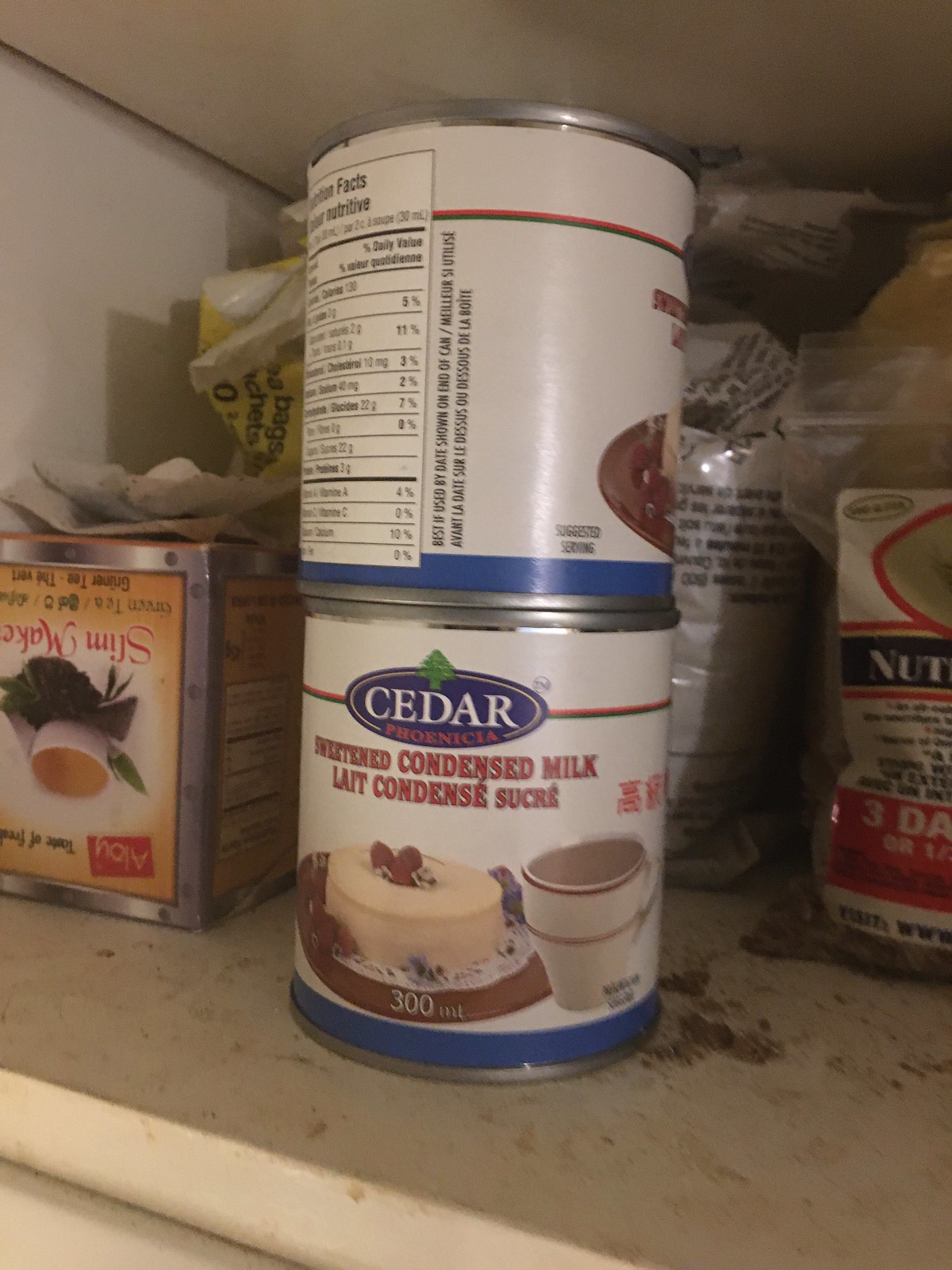The image is a slightly blurry, low-quality color snapshot of the inside of a kitchen cupboard, focusing on two stacked cans of Cedar brand sweetened condensed milk. The cans, which appear old, have a white label adorned with a blue strip at the bottom, depicting a piece of cake and a coffee cup. The bottom can's label, displaying the brand name "Cedar," faces the viewer, while the top can shows its nutrition facts. The shelving, made of worn and dirt-streaked white wood with peeling paint, forms the backdrop. To the left, an upside-down Slim Make tea box is visible, and various bags, possibly containing nuts, grains, or brown sugar, clutter the background, adding to the disorganized appearance.